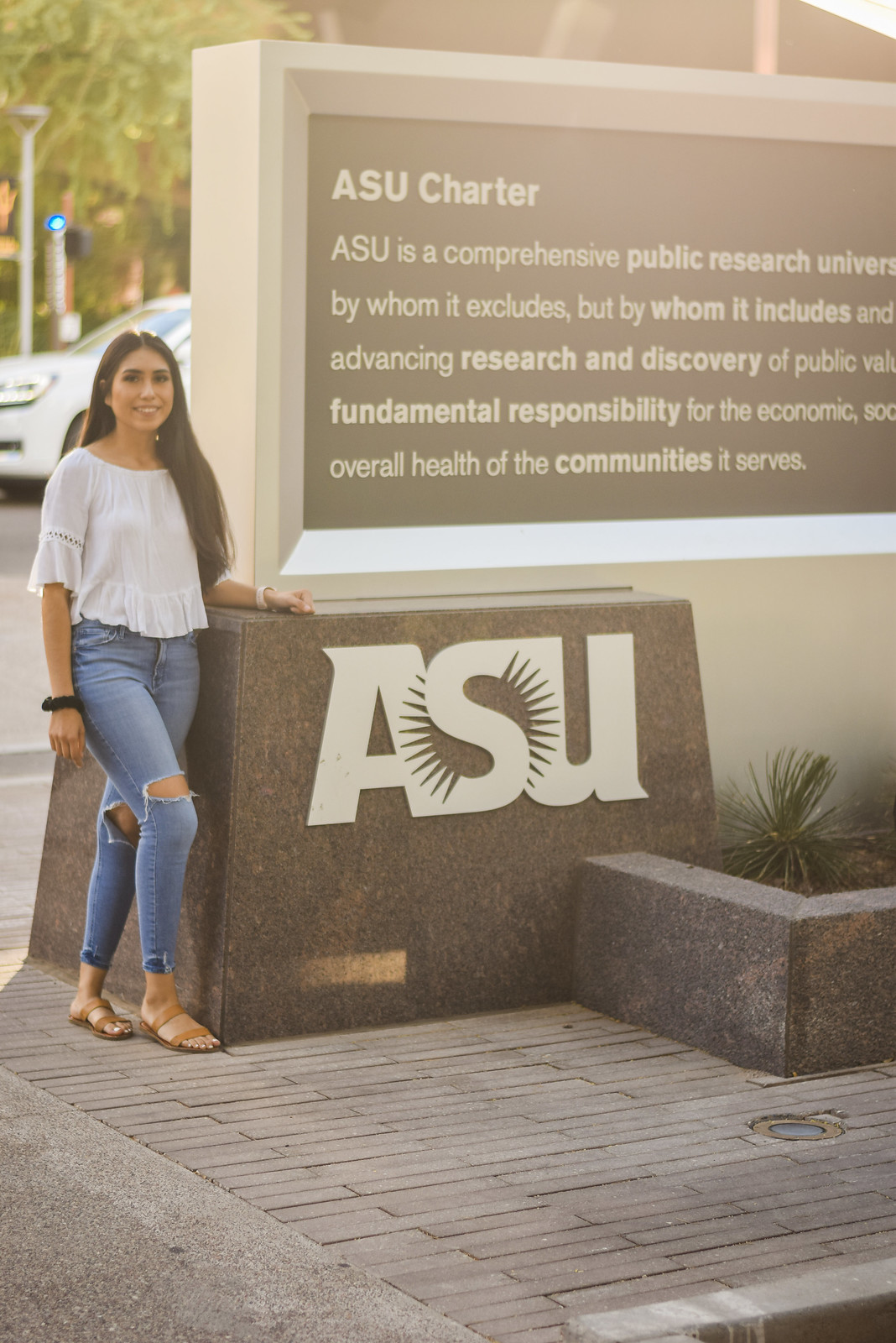A young woman with long brown hair, wearing a white shirt, ripped skinny blue jeans, and brown sandals, stands beside a stone sign bearing the words "ASU Charter." Her jeans feature rips above the right knee and on the left knee, and she has a hair tie on her right wrist. The sign, mounted on a concrete base, prominently displays "ASU" in white letters. Though partially obscured, the text mentions ASU as a comprehensive public research university, dedicated to inclusivity and advancing research and public value. In the background, there are glimpses of a car and a tree, portraying a clean and professional setting, possibly indicative of a promotional shot for the university. The overall scene exudes an academic atmosphere at Arizona State University.